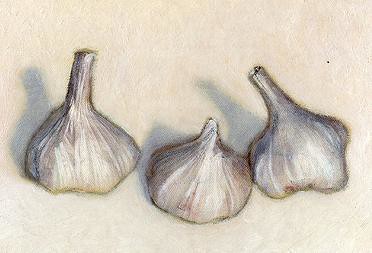This is a highly detailed, photorealistic illustration of three heads of garlic set against a textured cream-colored background. The drawing, not a photograph, vividly captures the fine details of the garlic skins, complete with grooves and subtle color variations ranging from white and gray to hints of purple and yellow. Positioned in a rectangular, landscape orientation, the garlic heads are arranged from left to right. The garlic on the left stands upright, featuring a tall stem and casting a shadow to its left. The middle garlic head sits slightly lower and more circular, with a shorter stem due to its angle. The rightmost garlic leans slightly against the central one, its stem pointing to the left and positioned higher in the image. Shadows from all three heads spread leftward, and the surfaces of each are distinctly bumpy, particularly the rightmost head. The detailed depiction, along with the rough texture of the background, creates a strikingly realistic representation of the garlic.